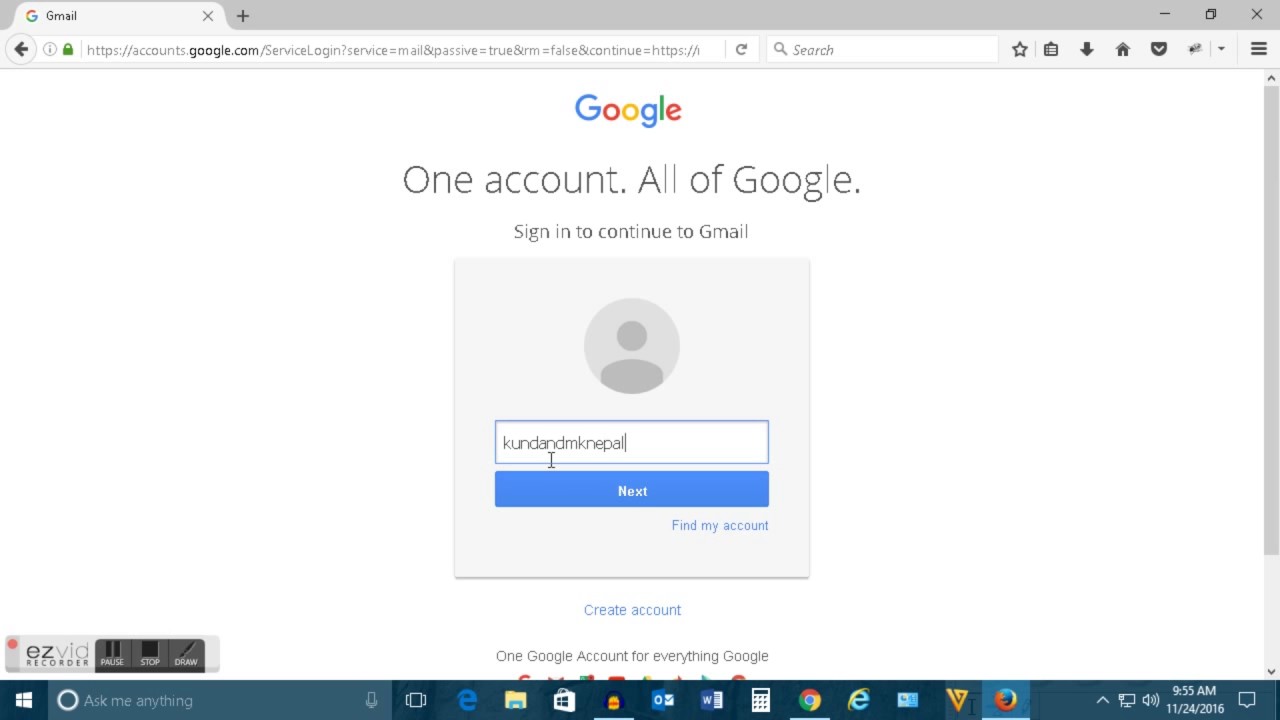The image depicts a Google login page open in a web browser tab, specifically at the URL accounts.google.com. Prominently featured at the top of the page is the Google logo, rendered in its signature colors: blue, red, yellow, and green. Underneath the logo, the text reads "One account. All of Google." Below this, the prompt states "Sign in to continue to Gmail." 

A light gray rectangular input field follows, which contains a circular icon of a person. In the data field, the username "KUNDANDMKNEPAL" is partially entered, with the cursor positioned after the "D" in "KUNDAN". 

Beneath this field is a blue button labeled "Next," and to the right of this button, the text "Find my account" is displayed in blue. Further down the page, outside the input box, there is an option "Create account" also in blue text. The footer text reads "One Google Account for everything Google."

On the left side of the screen, the Ezvid screen recorder interface is visible, showing controls for "Pause," "Stop," and "Draw." Additionally, a scrollbar on the right side of the page indicates that more content can be viewed by scrolling down.